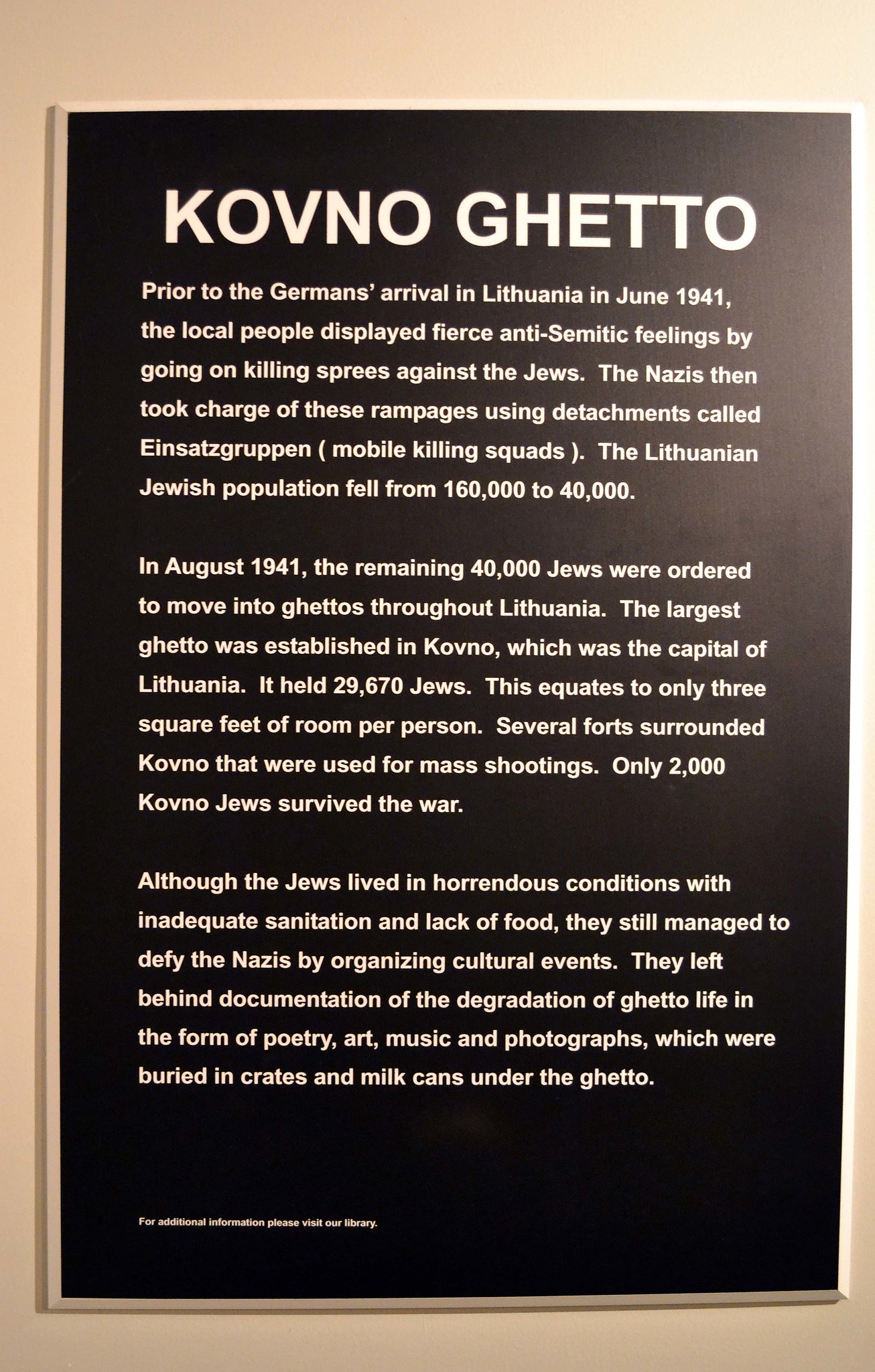The image shows an informative sign with a black background and white text, mounted on a yellowish-orange backdrop. The top of the sign prominently features the bold, capitalized words "Kovno Ghetto." It provides a detailed historical account, spread across three paragraphs, beginning with: "Prior to the Germans’ arrival in Lithuania in June 1941, the local people displayed fierce anti-Semitic feelings by going on killing sprees against the Jews. The Nazis then took charge of those rampages using detachments called Einsatzgruppen, or mobile killing squads. The Lithuanian Jewish population fell from 160,000 to 40,000." 

The second paragraph continues: "In August 1941, the remaining 40,000 Jews were ordered to move into ghettos throughout Lithuania. The largest ghetto was established in Kovno, the capital of Lithuania, which accommodated 29,670 Jews, equating to only three square feet of room per person. Several forts surrounded Kovno and were used for mass shootings. Only 2,000 of the Kovno Jews survived the war."

The final paragraph reads: "Although the Jews lived in horrendous conditions with inadequate sanitation and lack of food, they still managed to defy the Nazis by organizing cultural events. They documented the degradation of ghetto life through poetry, art, music, and photographs, which were buried in crates and milk cans under the ghetto." The sign is framed, and at the bottom left-hand corner, smaller white text begins with "For additional information, please," followed by three less legible words. The pinkish edges of the background, which aren't perfectly centered, frame the sign.